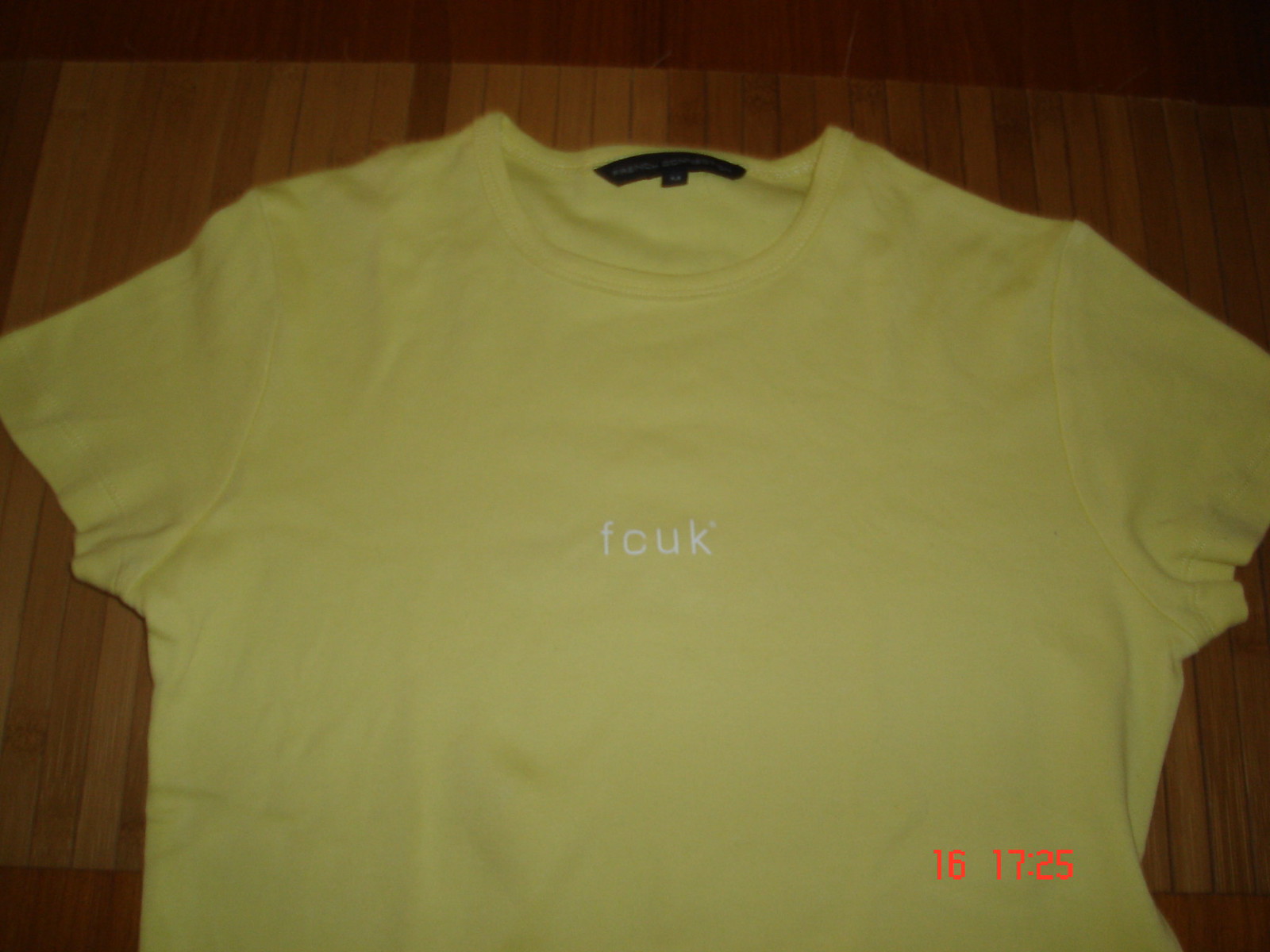This photograph features a white T-shirt that has become discolored over time, giving it a yellowed appearance. The image quality is poor, likely due to being taken with an old digital camera, resulting in bad lighting and a generally blurry aspect. The T-shirt prominently displays the letters "f-c-u-k," which seem to be a playful adaptation of a cuss word. At the bottom of the T-shirt, the numbers "16 17 25" are visible, though their significance is unclear. The background consists of thin, wooden planks, indicating the T-shirt is laid out on a table. Due to the image being out of focus, the brand label is not discernible, but it appears to have a black tag.